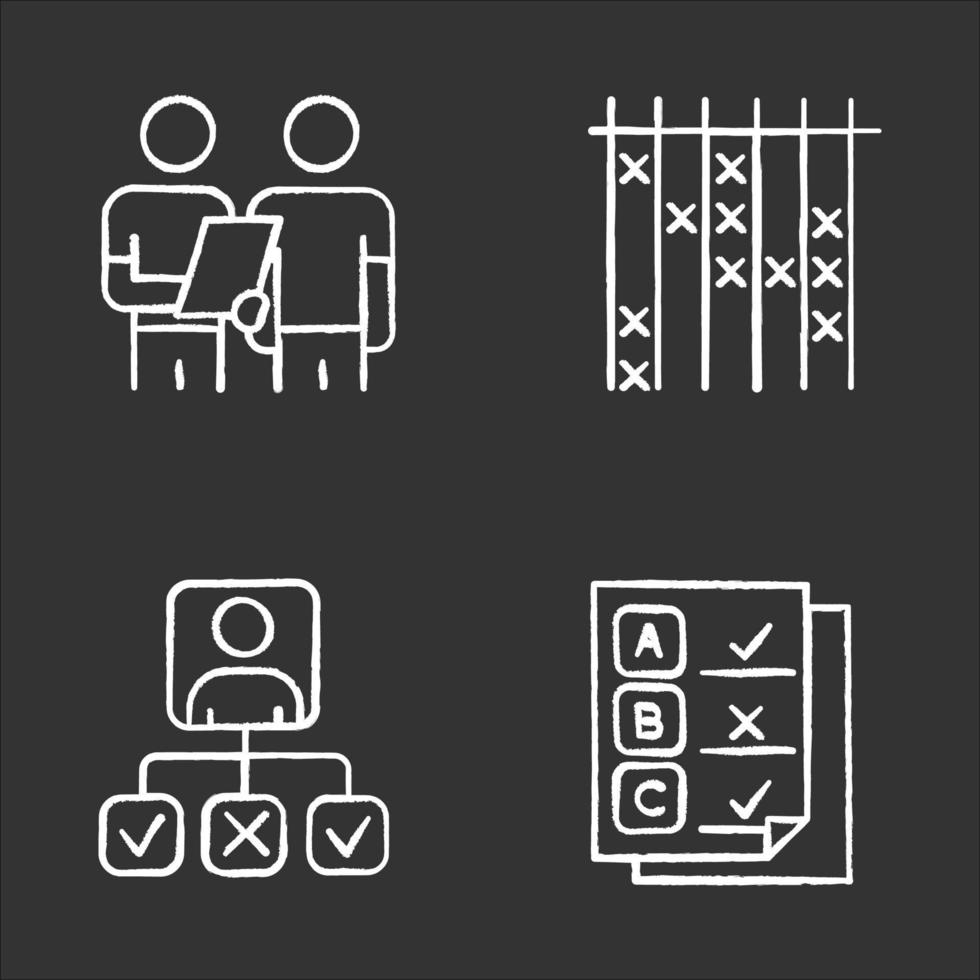This black-and-white infographic, likely designed for an informational website or educational context, features a square layout with a solid black background and white line art illustrations. Arranged in a 2x2 grid format, each section contains specific visual elements:

- **Top Left**: Two stick-figure men, dressed in t-shirts, are standing side by side with one holding a document—possibly a clapboard. They appear to be engaged in a discussion.
- **Top Right**: A grid resembling a tic-tac-toe board, formed by a horizontal line at the top and six vertical lines creating five columns. Each column contains various X's, suggesting a checklist or planning tool.
- **Bottom Left**: A stick figure within a box, potentially a computer screen. Below this figure is a flowchart with arrows pointing downward to three smaller boxes containing a checkmark, an X, and another checkmark respectively.
- **Bottom Right**: Two overlapping, letter-sized documents, with the top document showing "A, B, C" vertically aligned on the left. Adjacent to these letters are a checkmark by A, an X by B, and a checkmark by C.

This detailed graphic clearly conveys a structured, educational theme through its institutional stick-figure style.